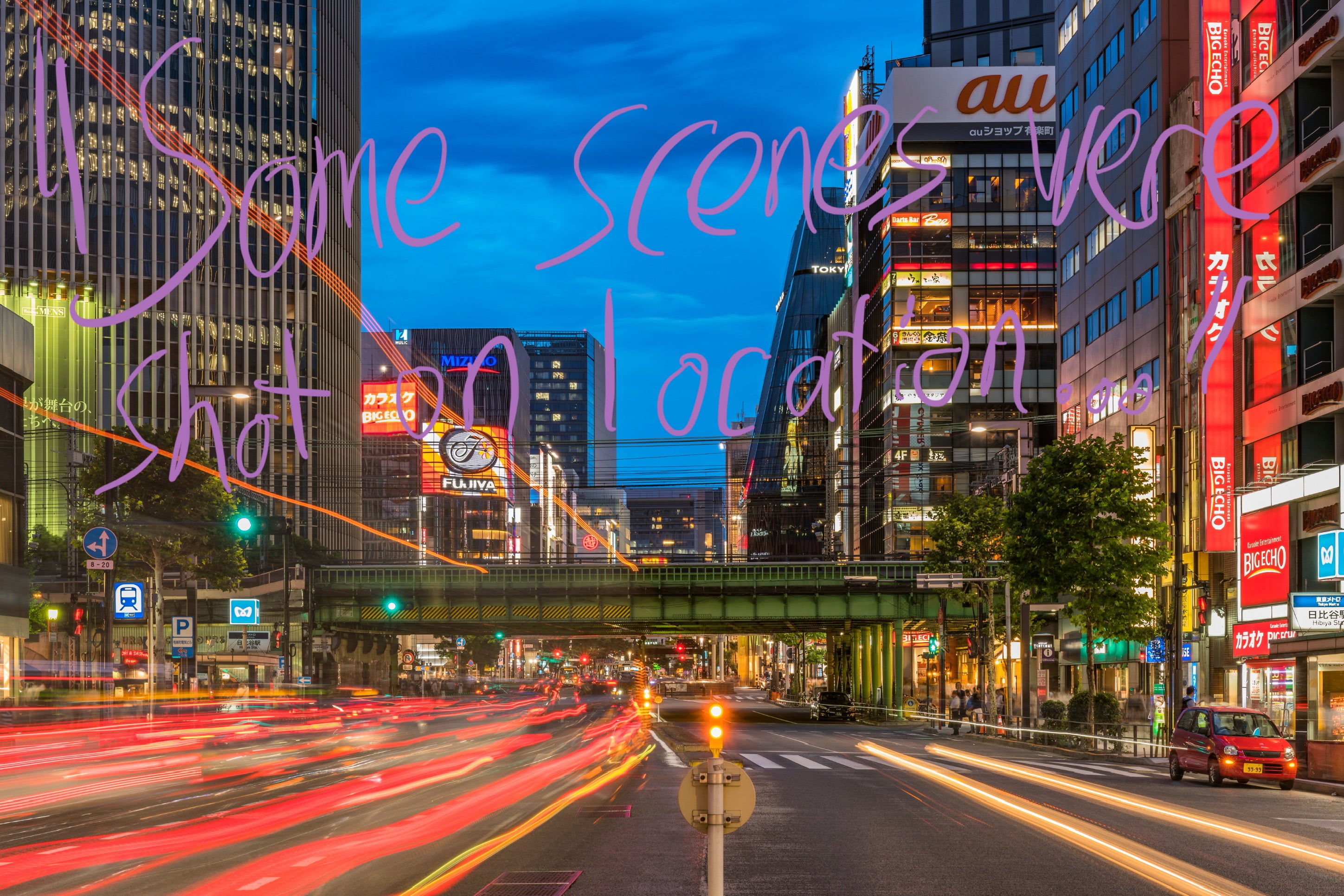This captivating photograph depicts a bustling urban setting as night falls, with a darkening sky transitioning from deep blue at the top to a slightly lighter hue near the horizon. The scene is framed by towering city buildings on both sides, their interior lights illuminating the growing darkness. The wide street, likely with six lanes, stretches towards the horizon, where a bridge connects the left and right sides, creating a visual anchor in the background. 

On the left side of the street, the taillights of cars create a red blur, hinting at the city's constant motion, captured with a slow shutter speed for a dynamic effect. In contrast, the right side of the road appears quieter, with a solitary, small red car parked along the curb. Brightly lit signs and neon lights, especially on the buildings to the right, suggest a vibrant nightlife, possibly in Tokyo or another Japanese city, as indicated by the distinct lettering on the signage. 

Overlaid on the image in purple text at the top, the phrase, "For some scenes were shot on location," adds a touch of intrigue, as if lifting a curtain on a cinematic moment frozen in time. The combination of blurred taillights, bright signs, and a sky in transition provides a striking visual narrative of urban life at dusk.